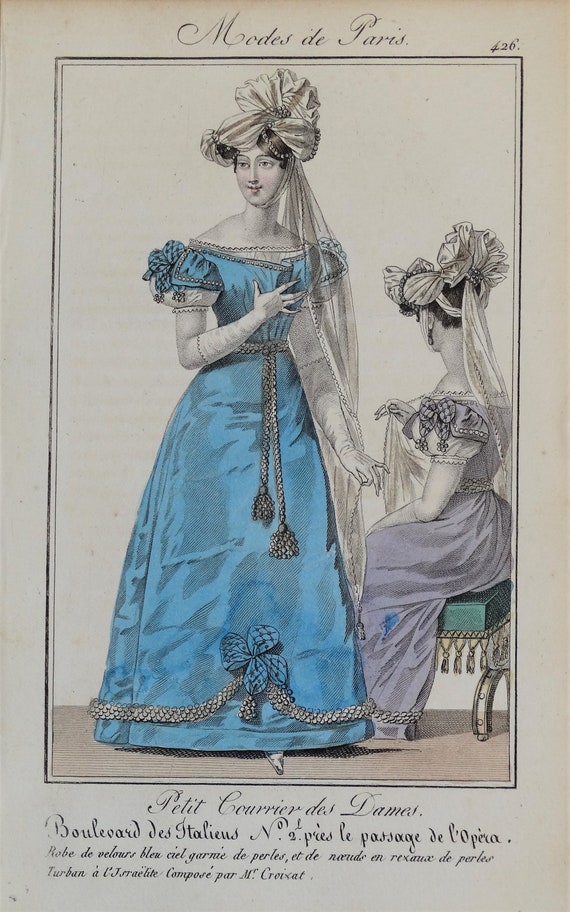The image is a vintage-style advertisement card, likely from a magazine, with a faint grayish, off-white cream background and black-and-white illustrations accented with color. The card is titled "Modes de Paris" at the top, indicating it's a French advertisement for fashion. The scene features two women in Victorian-era gowns.

The woman on the left, who is standing, wears a large white bonnet and white gloves. Her sky-blue dress has prominent poofy shoulders, an empire waistline accentuated with a rope-style sash, and a similar roping trim at the bottom, highlighted by a blue bow at the center. Her right hand rests on her chest while her left arm hangs down.

To her right, a second woman is seated on a stool with a green cushion. She wears a lilac-colored dress with similarly ornate poofy sleeves, white gloves, and a white bonnet. Her dress also includes a blue bow with black dots. She is turned away, showing the back of her head and neck, with her shoulders exposed.

The text at the bottom of the image reads "Boulevard des Italiens," suggesting its Parisian context and possible location reference. The entire scene is framed by a thin black line, adding a formal touch to the advertisement.